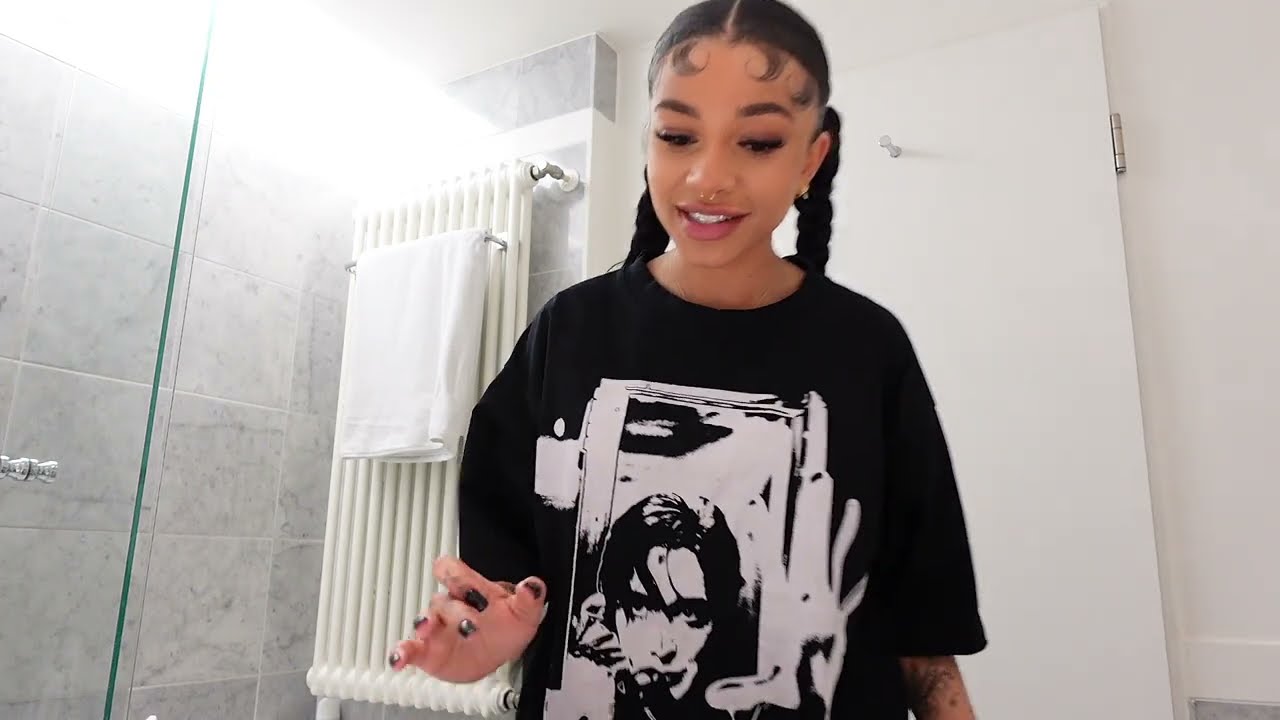The image showcases a young African-American woman with straight, dark black hair styled into two braids hanging behind her back. She is standing in a predominantly white bathroom, possibly a hotel, due to the neatly wrapped towels and a towel warming rack with a metal bar. The bathroom has features like a clear shower door with a chrome handle, gray tile or granite squares, and a door with a hook on the right side.

The woman stands center with her right arm down and her left arm bent at the elbow, holding her phone. She has heavy makeup, black fingernail polish, tattoos visible on her arm, and a nose ring. She is dressed in a black t-shirt adorned with an image of a man holding his hand out, possibly a singer. The setting and composition of the photo give it the appearance of a social media post.